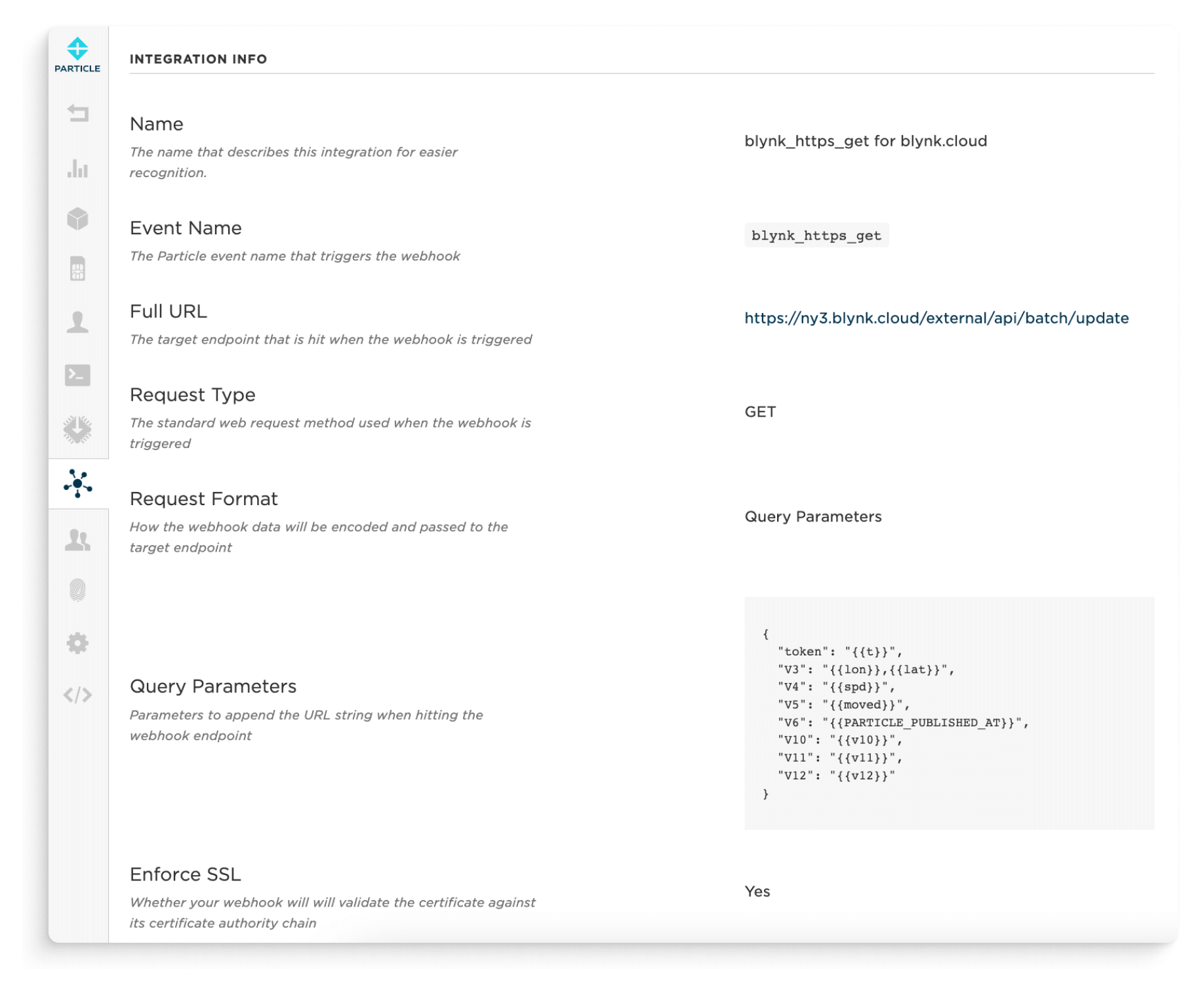A screenshot of a computer screen displaying an integration setup page. On the left, a slim gray sidebar extends vertically, featuring various action icons. The top of the main content area is labeled "Integration Info" with a horizontal line beneath it. Below, the page is divided into two main columns. The left column lists descriptive labels:

- **Name**: Describes this integration for easier recognition.
- **Address**: Displays an HTTP address relevant to the integration.
- **VIN Name**: A particular VIN name that triggers the webhook, with an associated HTTP address.
- **URL**: Specifies the target endpoint hit when the webhook is triggered, accompanied by an HTTP address.
- **Request Type**: The standard web request method used when the webhook is triggered.
- **Request Format**: How the webhook data will be encoded and passed to the target endpoint.
- **Query Parameters**: Additional parameters to append to the URL string when hitting the webhook endpoint.
- **Enforce SSL**: Located at the bottom.

The right column displays the corresponding details, mainly HTTP addresses, for each label in the left column, providing comprehensive information about the integration's setup and functionality.